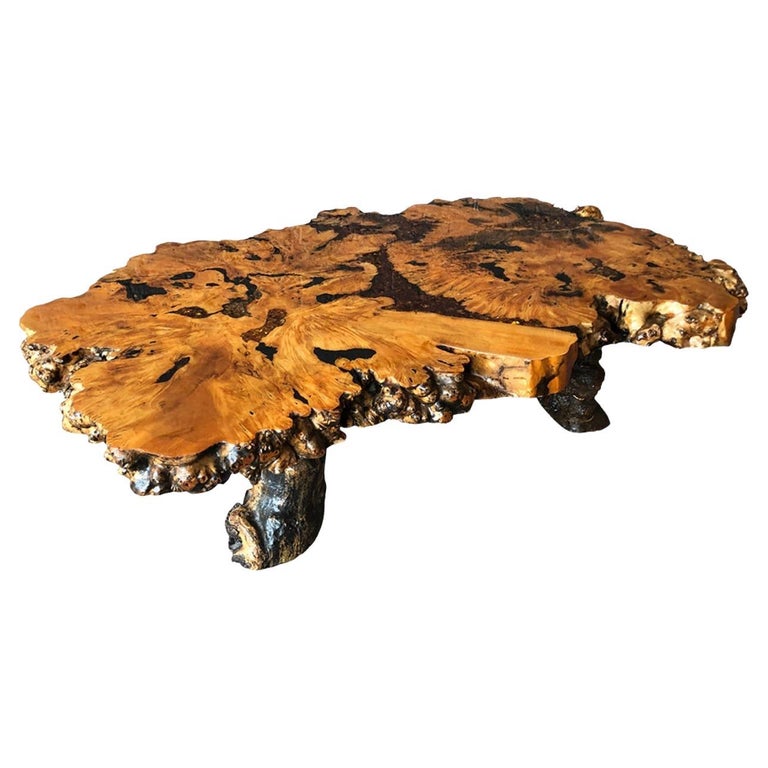The image showcases a meticulously handcrafted wooden coffee table set against a stark white background. The tabletop appears to have been carved from a single, thick tree trunk, with intricate designs and natural patterns that suggest a blend of artistic carving and possible assembly of various wood pieces. The surface has hues of light orange, brown, and faint green stains, with darker and lighter patches along the edges. Noteworthy are the blackened sections indicating potential burning techniques employed during creation. The table features raw, natural edges and legs that retain the bark from the original tree, emphasizing its rustic and organic aesthetic. The polished wood grain reveals a smooth finish, highlighting the unique, natural variants inherent in the wood.